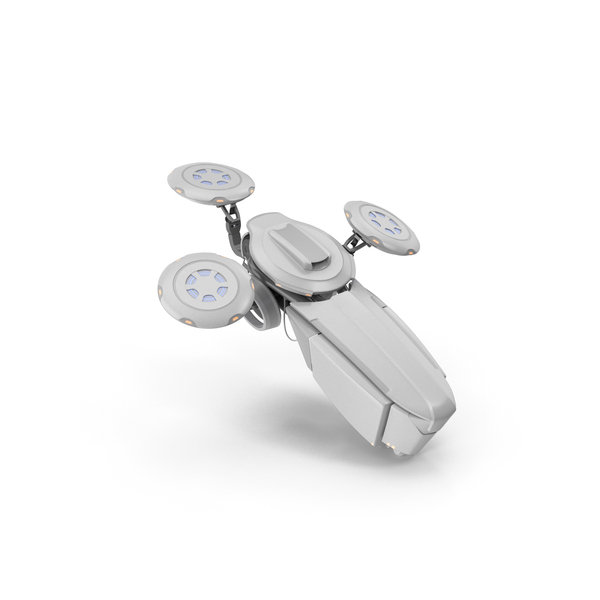The image depicts a sleek, white, futuristic-looking exercise device or model, reminiscent of a spaceship. Its body is primarily white, with a blend of oval and rectangular shapes, creating an undefined silhouette. The central structure of the device slopes upwards to the left, starting from a rounded back positioned at the bottom right of the image. This back section appears to be the main point of contact with the surface.

Prominently featured are three circular pods at the front of the device, each adorned with what seem to be orange lights around their sides. These pods possibly function as pedals or components of the device, hinting at an exercise-related purpose. Each pod has a gear-like design in its center, with a strap connecting the middle piece to the left pod, looping underneath the device.

Above the central body, there is a distinctive round disc with a protruding rectangular outcrop, bordered by silver and capped with a darker gray top. This disc is accompanied by another circular feature intersecting between the pods, adding to the complexity of the design. The top of the circular parts showcases spokes, resembling the shape of a wheel. 

The entire model sits against a stark white backdrop, enhancing its futuristic aesthetic. Small metallic components and light blue accents seen underneath add to its high-tech appearance, making it resemble an advanced piece of technology or a conceptual spacecraft model.